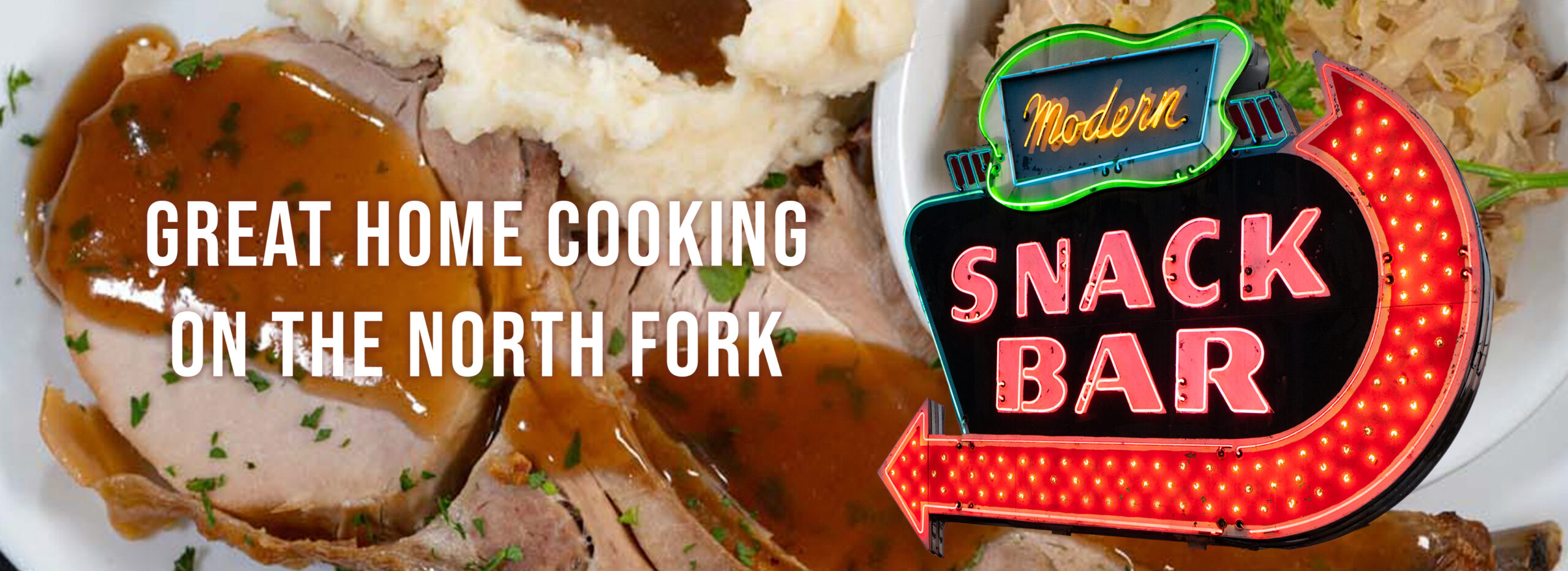This web advertisement for the restaurant Modern Snack Bar showcases a tempting plate of food as its central visual element. The image, taken from directly overhead, features a serving of pork slices garnished with chopped parsley and coated in brown gravy, accompanied by a generous helping of mashed potatoes, also topped with gravy. To the right, a white ramekin contains what appears to be fried onions, possibly sauerkraut, and garnished with a sprig of parsley.

Overlaying the food is the vibrant Modern Snack Bar logo, which adds a retro flair reminiscent of neon diner signs. The word "Modern" is prominently displayed in bold yellow script, encased within a blue trapezoid and surrounded by a green squiggly line. Below it, "SNACK BAR" is written in all caps with pink neon letters on a black rectangular background. A sweeping red illuminated arrow wraps from the top right, around the right edge, and across the bottom, directing attention to the tagline.

The tagline "Great Home Cooking on the North Fork" is elegantly superimposed over the pork chops and mashed potatoes, emphasizing the restaurant's appeal. The sleek, eye-catching design of the ad, along with its vibrant colors and detailed depiction of the meal, effectively highlights the homey yet modern dining experience offered by Modern Snack Bar.